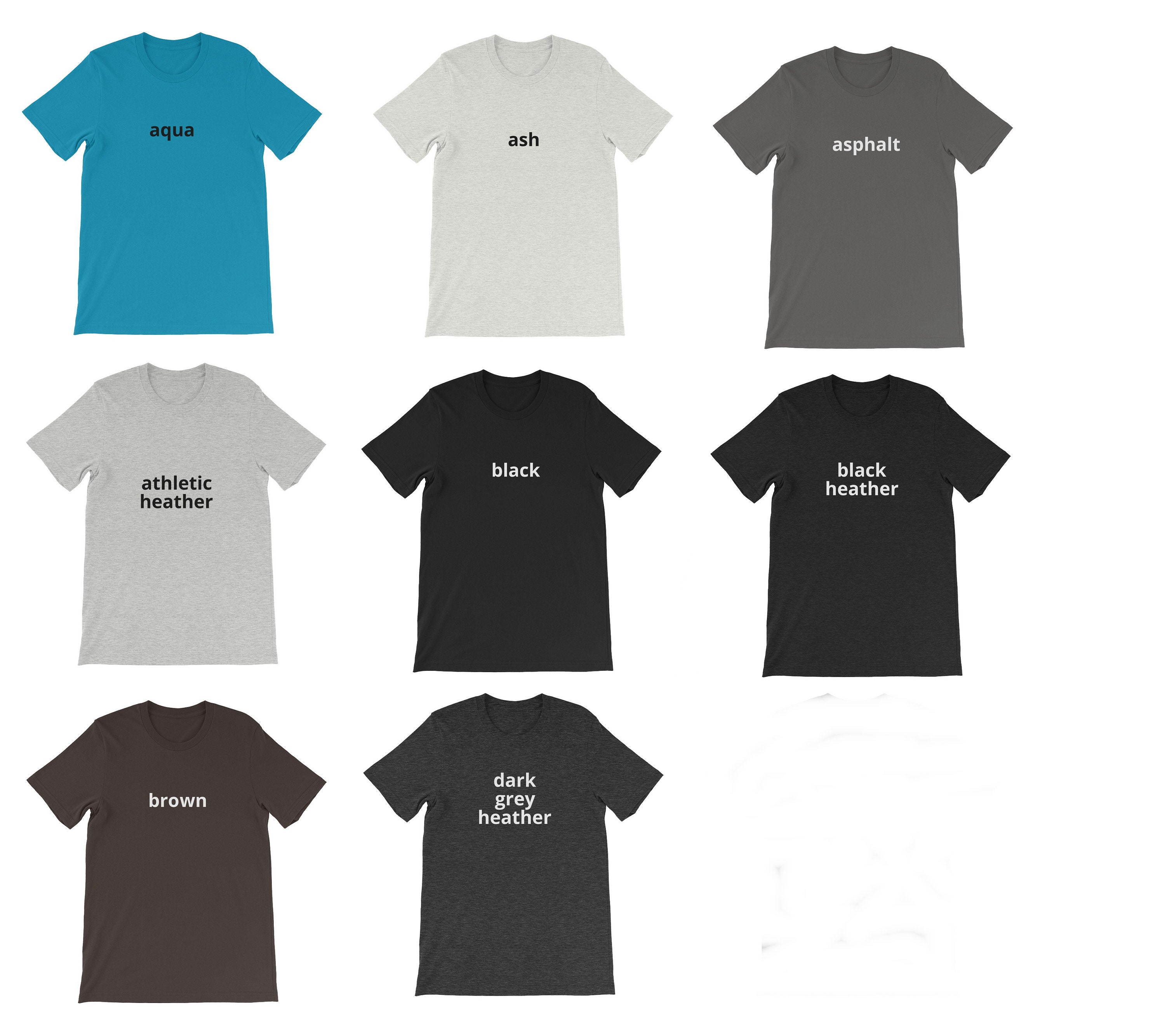The image features a collection of eight unisex t-shirts displayed as if on a retail website. Each shirt, predominantly of a u-neck design with short sleeves, is distinctly colored and labeled. The first shirt is labeled "Aqua," showcasing an aqua blue hue, albeit with a resemblance closer to cerulean. Notably, there are small wrinkles near the left sleeve and three wrinkles near the bottom. 

Next is a shirt labeled "Ash Gray," which appears almost white, followed by "Asphalt," a darker gray shade. Below these, there is an "Athletic Heather" shirt, characterized by its gym uniform-like Heather gray fabric. Centrally located is a solid black shirt and adjacent to it is a "Black Heather" shirt. 

Beneath the "Athletic Heather" shirt is a brown-colored shirt. Completing the lineup is the "Dark Gray Heather" shirt, a darker variant of the Heather style. The image illustrates the t-shirts in a lifelike manner, accentuating even minor details such as fabric wrinkles.